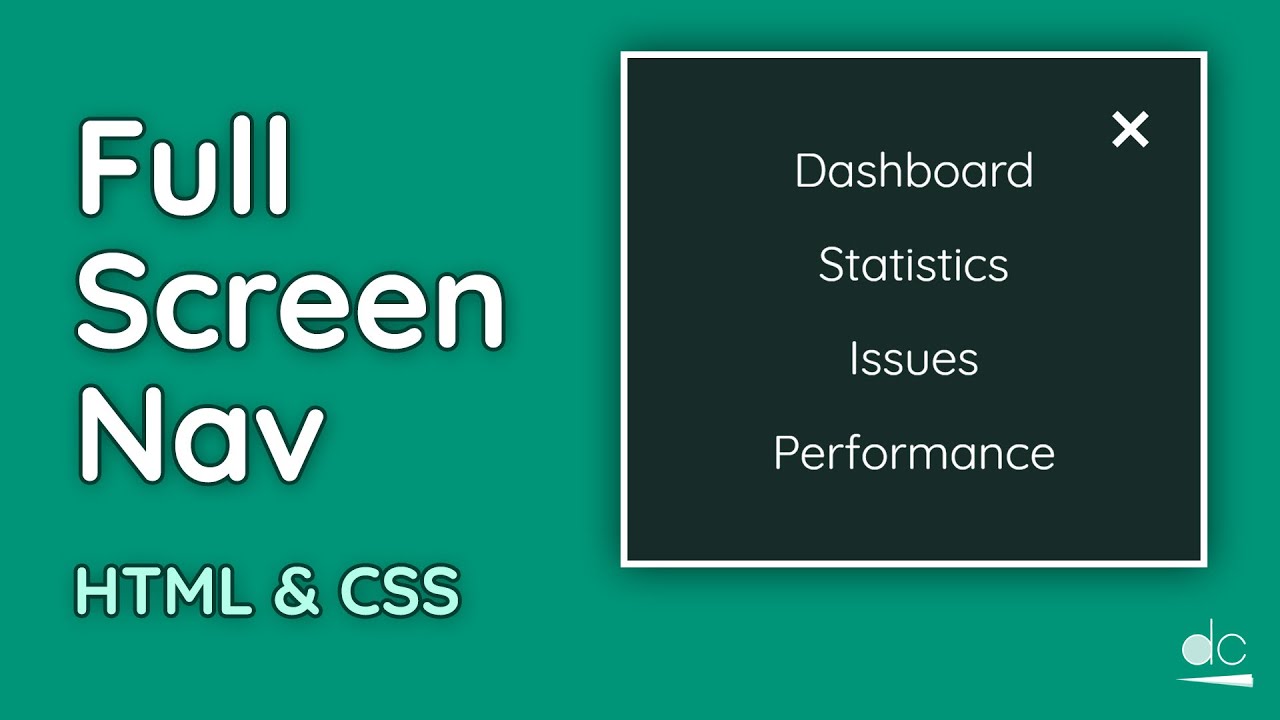This image features a solid green background. On the right half, there's a vertically oriented, dark green shaded square. Positioned at the top right inside the square is an "X," drawn in white, to indicate a close button. 

Inside this square, the text, drawn in white, is displayed in four distinct sections:
1. Dashboard 
2. Statistics 
3. Issues
4. Performance

Each section is placed vertically below the previous one, in the order mentioned.

To the left of the square, still within the green background, the text "Full Screen Nav" is written in white.

At the bottom of the image, in slightly lighter green text, are the words "HTML" and "CSS." 

Located at the bottom right corner, there's a gray-outlined icon featuring the letters "DC." Adjacent to "DC," there is a white paper plane icon facing towards the left, and below "DC," there's a lock icon.